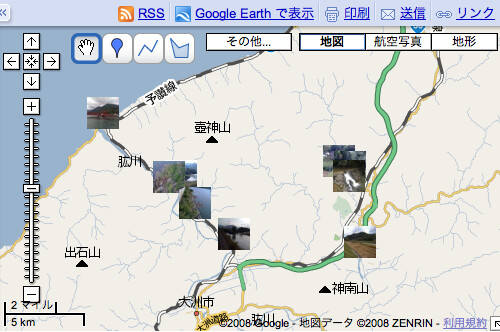The image depicts a screenshot from what appears to be an older version of a map application, potentially Google Earth, dated 2008 with a copyright to Zenrin. The interface includes various navigational tools and scales on the left side, such as arrows for directing views in any cardinal direction, a plus and minus zoom scale, and a kilometer distance scale. In the center, the map is labeled in Japanese kanji, highlighting a coastal region with rivers or streams. A light green path traverses the map along with various highways. Scattered across the map are small photos marking different landmarks and tourist attractions. Additional options for sharing, printing, and emailing can be seen at the top of the interface. The scene combines detailed geographical features with cultural elements, reflecting a mapped area somewhere in Japan.